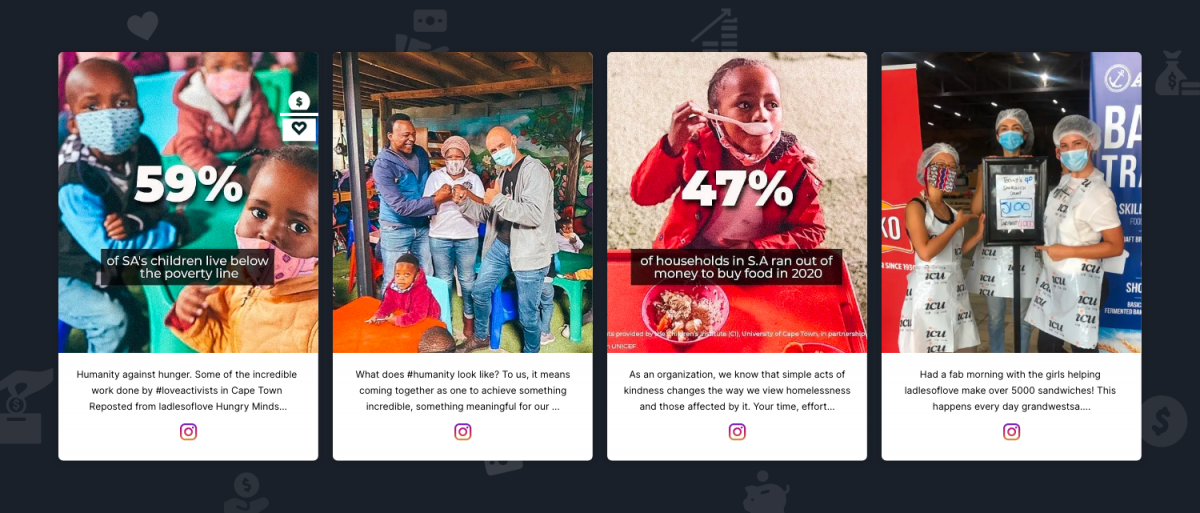This image features a screenshot from a website with a black background adorned with minimal graphics, including hearts, circular dollar signs, and a piggy bank with a coin being inserted. The primary focus of the image is a series of four panels, each showcasing images of people and impactful messages.

1. The first panel highlights a group of children with the caption: "Humanity Against Hunger. Some of the incredible work done by #LoveActivists in Cape Town, reposted by Ladies of Love Hungry Minds. 59% of South Africa's children live below the poverty line."

2. The second panel features three adults and some children with the message: "What does #Humanity look like? To us, it means coming together as one to achieve something incredible and meaningful..."

3. The third panel shows a child eating with the text: "47% of households in South Africa ran out of money to buy food in 2020. As an organization, we believe that simple acts of kindness can change the way we view homelessness and those affected by it. Your time, effort..."

4. The final panel presents three individuals wearing masks, accompanied by the statement: "Had a fab morning with the girls helping Ladies of Love make over 5,000 sandwiches. This happens every day. #GrandWestSA..."

Each caption underscores the pressing issues of poverty, hunger, and homelessness in South Africa, while also emphasizing community efforts and kindness in addressing these challenges.